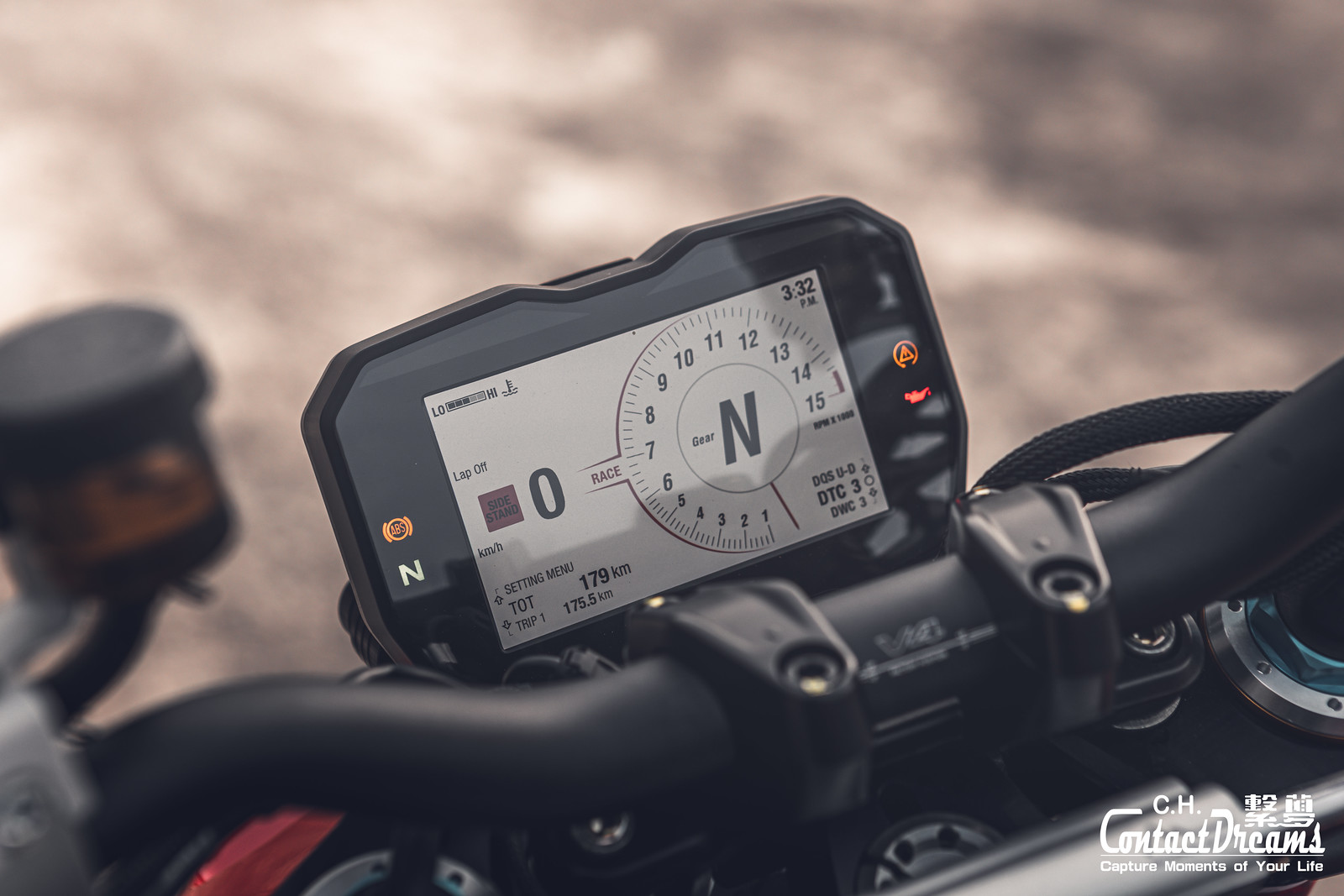A close-up shot of a digital display mounted on the black metal handlebars of a motorcycle, seemingly taken outdoors on a sunlit, dirt path. The display is square with a light gray background, slightly tilted to the left. In the center, it prominently features a circular speedometer, marked incrementally from 1 to 6, with wider gaps leading up to 15. "GEAR" and the letter "N" are centered within the circle, indicating the bike is in neutral. In the upper right corner, the time reads 3:32 PM, and "LO" is displayed in the far upper left corner. The display also includes a battery indicator with three lights and the text "LAPOFF" beneath it. Below the speedometer, a brown square with a large zero next to it displays "RACE," with "KM/H" right underneath. Further details include "SETTINGS MENU," "TAUT," 179 kilometers and 175.5 kilometers listed towards the bottom. The instrument panel features several indicator lights, including amber-colored lights and a green light with a capital "N", as well as an ABS warning light, an oil warning light, and a traction control light. The image, marked with a watermark in the bottom right corner, states "CH Contact Dreams Capture Moments of Your Life." The blurred background hints at a dirt path, emphasizing the off-road setting.